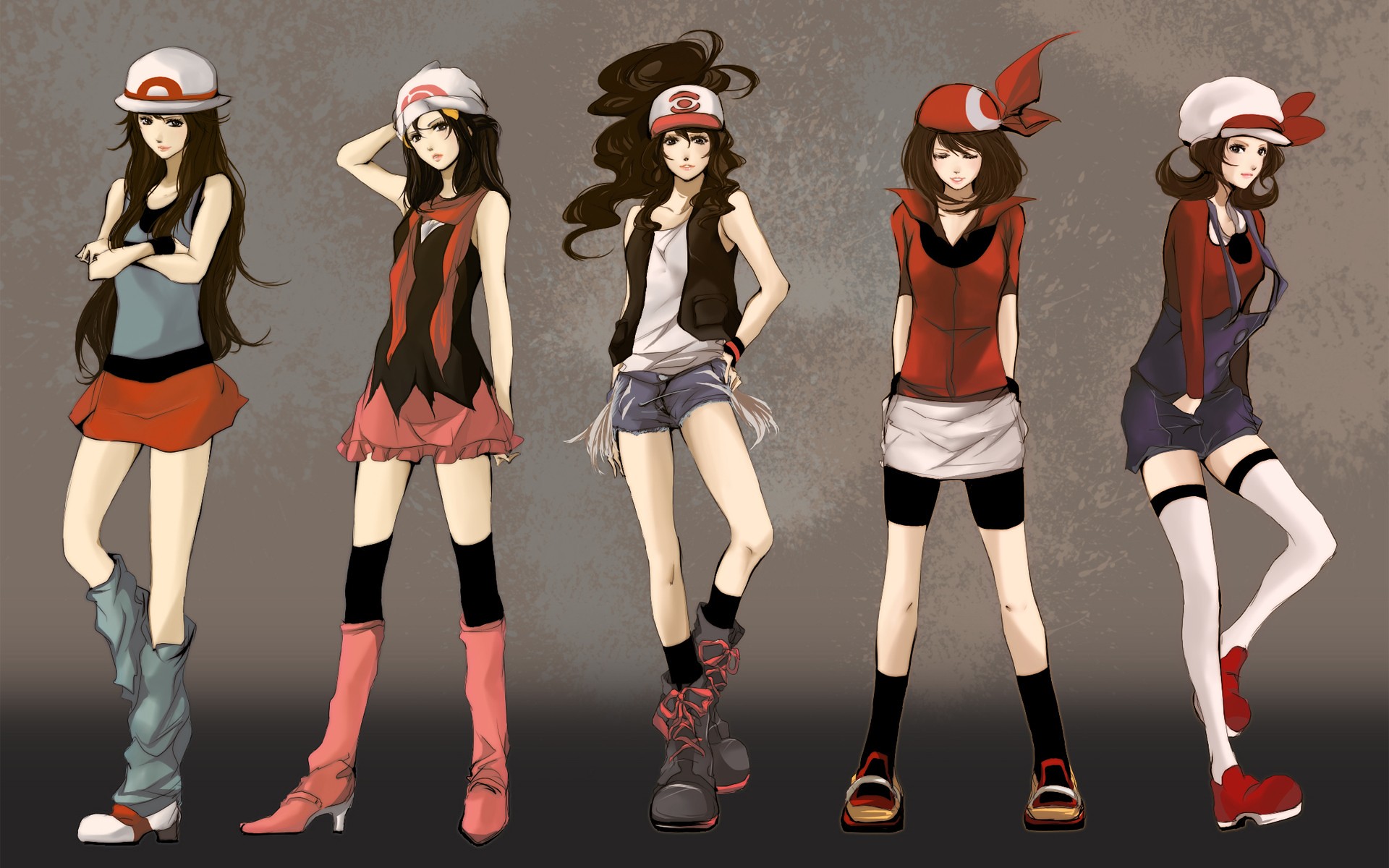The image depicts a group of five cartoonish, anime-style women standing in various poses against a textured grey background that fades into a darker feathered grey at the bottom. Each woman has long dark hair and wears a distinct outfit, featuring common elements of hats, thigh-high socks, and either skirts or shorts. The first woman wears a red and white hat, a gray shirt paired with a red skirt, and long gray leg warmers with red and white shoes. The second woman is dressed in a black and white dress with a matching white hat, knee-high black socks, and red boots. The third woman sports a vest, a short shirt, and shorts with combat boots. The fourth woman has a red vest with a high collar and a red hat adorned with a bow, white shorts over black shorts, sandals, and black socks. The fifth woman wears a white hat with a bow, overalls, thigh-high stockings, and red boots. Their outfits incorporate shades of red, black, white, and hints of blue, and they strike various poses, including arms crossed, hand behind the head, hands on hips, and hands in pockets.